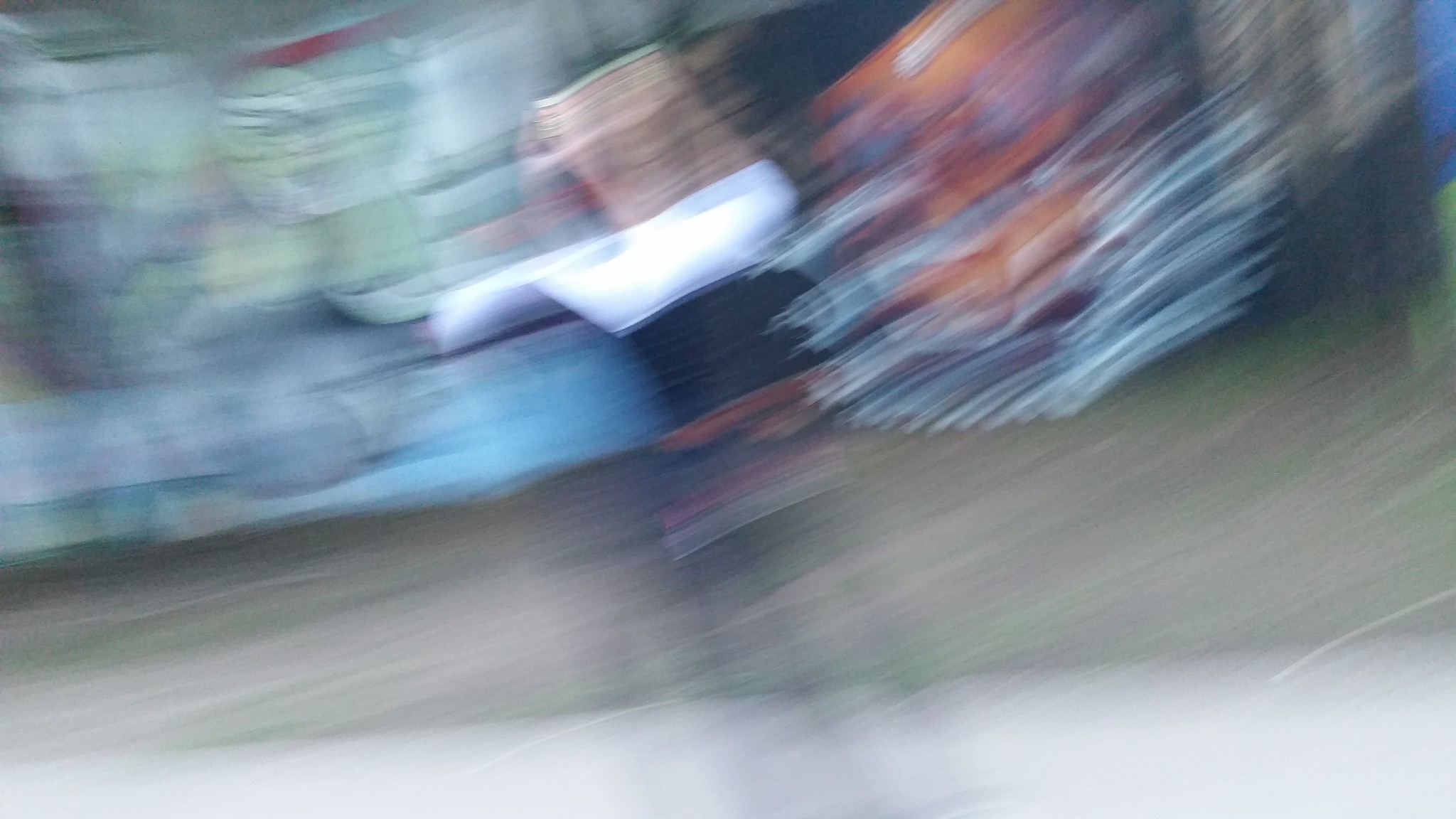In this photograph, a girl stands at the center amidst an indistinct background due to significant motion blur, indicating that the photographer was in rapid movement while capturing the image. The photo’s low resolution obscures precise details, but it appears that the setting features walls adorned with vibrant graffiti. The graffiti, a mix of colors including green, blue, orange, and white, creates a colorful yet unclear backdrop. The girl's attire seems to include a white shirt, possibly layered with a black corset, though the motion blur makes this challenging to confirm.